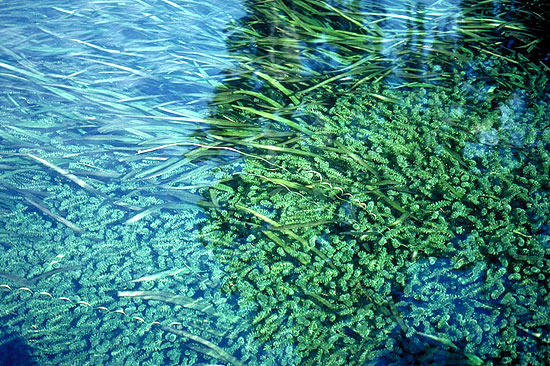The image is a highly detailed, close-up photograph of a still pond, focusing on the underwater and partially protruding vegetation. Dominated by shades of light and dark green, the photograph showcases tightly packed pond grass, with the darker green fronds extending above the water's surface while the lighter green fronds remain submerged. The scene is devoid of wildlife, and the tranquil water shows no sign of movement or disturbance, captured with bright outdoor lighting and in sharp focus. The right side of the image is primarily occupied by the emergent fronds, while the left side is filled with submerged vegetation. There's an intriguing piece of curled, possibly dead seaweed floating in the center, emphasizing the intricate interplay between the various plant life forms. The overall composition features a mix of long, straight grass and shorter, coiled seaweed, suggesting a vibrant yet serene aquatic ecosystem.